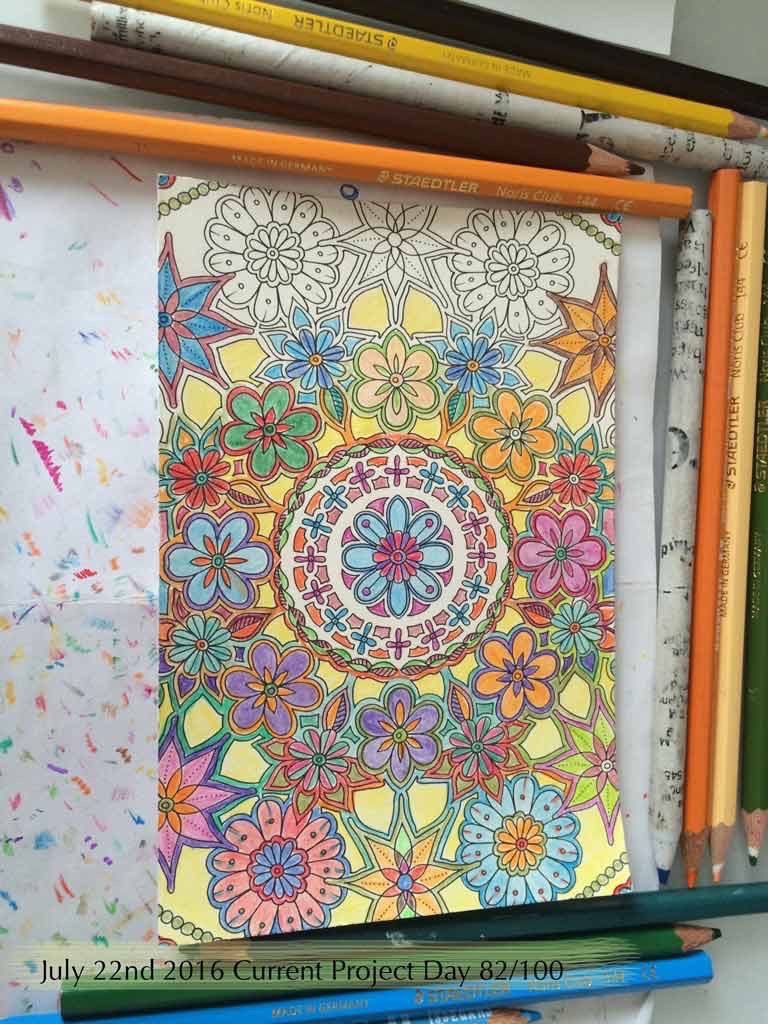This detailed image shows an 80-85% completed adult coloring page featuring a central mandala surrounded by various symmetrical floral designs, including six-petaled flowers and simple geometric shapes. The vibrant artwork is colored with a range of colored pencils, predominantly yellow, but including green, pink, blue, orange, purple, and black hues. The background for the central medallion is yellow, while the mandala and flowers are meticulously colored in. Pencils are laid horizontally across the top edge and perpendicularly on the right side of the image, with notable colors being green, blue, yellow, and orange. Several flowers and a star-shaped figure at the top remain uncolored, indicating the work in progress. At the bottom, the text "July 22, 2016, current project day, 82 out of 100" is inscribed in black typewritten letters, over a green and blue pencil backdrop. A white scratch pad with multicolor splotches from testing the pencils lies nearby, adding a practical touch of the artist’s process.